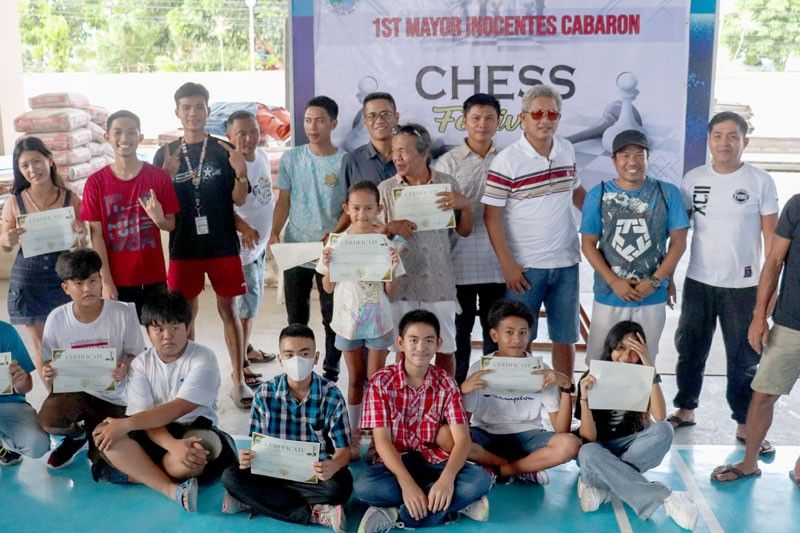A large group of people, predominantly composed of children, are posed for a group photo in front of a large sign with a blue border featuring the word "chess" and an image of a pawn. The top of the sign also reads "First Mayor Innocentes Cabaron" in red letters. The group includes 15 to 18 individuals, many of whom are smiling and holding certificates, indicative of a chess tournament. The front row of six to seven children includes a boy wearing a white surgical mask. Behind them, taller, older children and some adults are visible, including a man in white with red sunglasses, a light blue shorts and two other adults around his age. The backdrop reveals trees on both sides, and everyone is seated on a blue floor, with one particularly small girl holding her certificate prominently in the middle row. The overall atmosphere is celebratory and joyful.